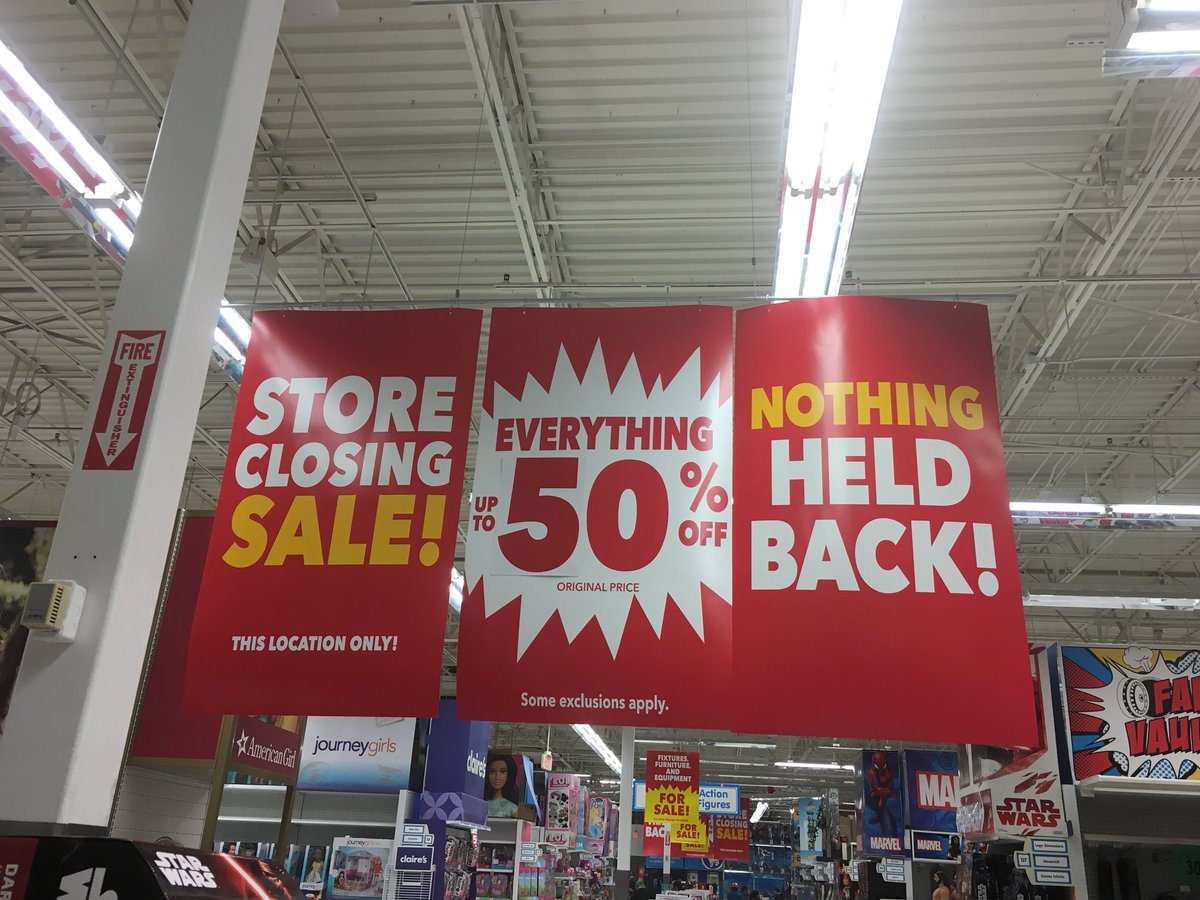This photograph captures the interior of a retail store, showcasing a unique perspective from the ground up. Dominating the image is the store's ceiling, which occupies a significant portion of the visual frame. Hanging prominently from the ceiling are three large, eye-catching red signs.

On the right, one sign declares in bold white font, "STORE CLOSING," followed by a smaller note, "Sale," and a further clarification, "This Location Only."

The central sign grabs attention with a white starburst shape containing the text, "EVERYTHING UP TO 50% OFF ORIGINAL PRICE," with a disclaimer underneath that reads, "Some Exclusions Apply."

The leftmost sign, located on the right side of the image, confidently states, "NOTHING HELD BACK."

This visual detail underscores the store's significant markdowns and closing sale, providing a sense of urgency to potential shoppers.